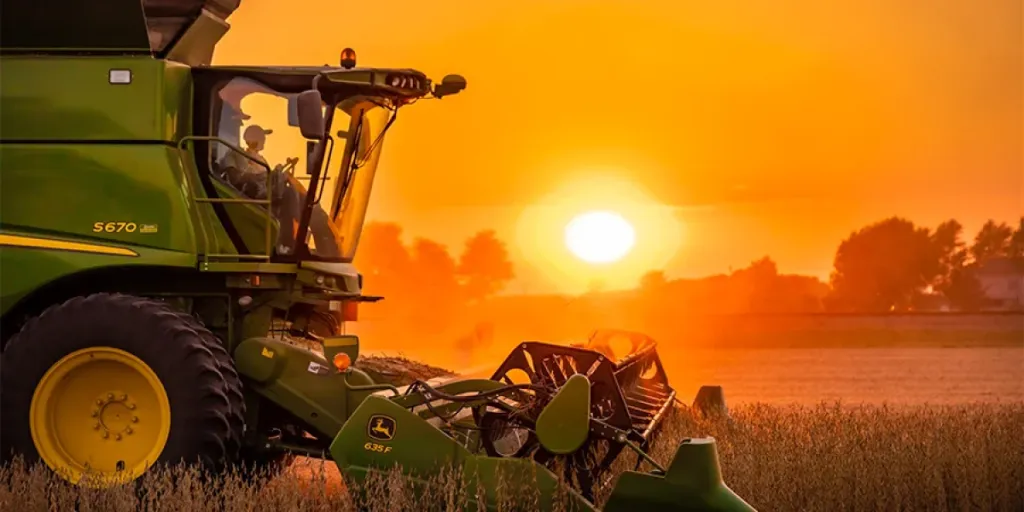The image portrays a meticulously detailed, photorealistic illustration of a large, modern green John Deere S670 tractor with an emblematic yellow leaping deer logo. The enormous black tires have thick treads and yellow hubs. The tractor, equipped with a long arm bearing a spike-like cylinder, is either plowing a field of wheat or rolling over some hay. The vehicle features a spacious front cabin with large glass doors, providing a clear vantage point for the farmer inside, who is wearing a ball cap and gazing toward the horizon. The vibrant background showcases a golden, peachy sky illuminated by a giant ball of light, likely the sun either rising or setting, casting its glow over distant shadows of houses and trees in a vast green field. The entire scene is awash in warm hues of yellow, orange, and red, emphasizing the serene, rural landscape.